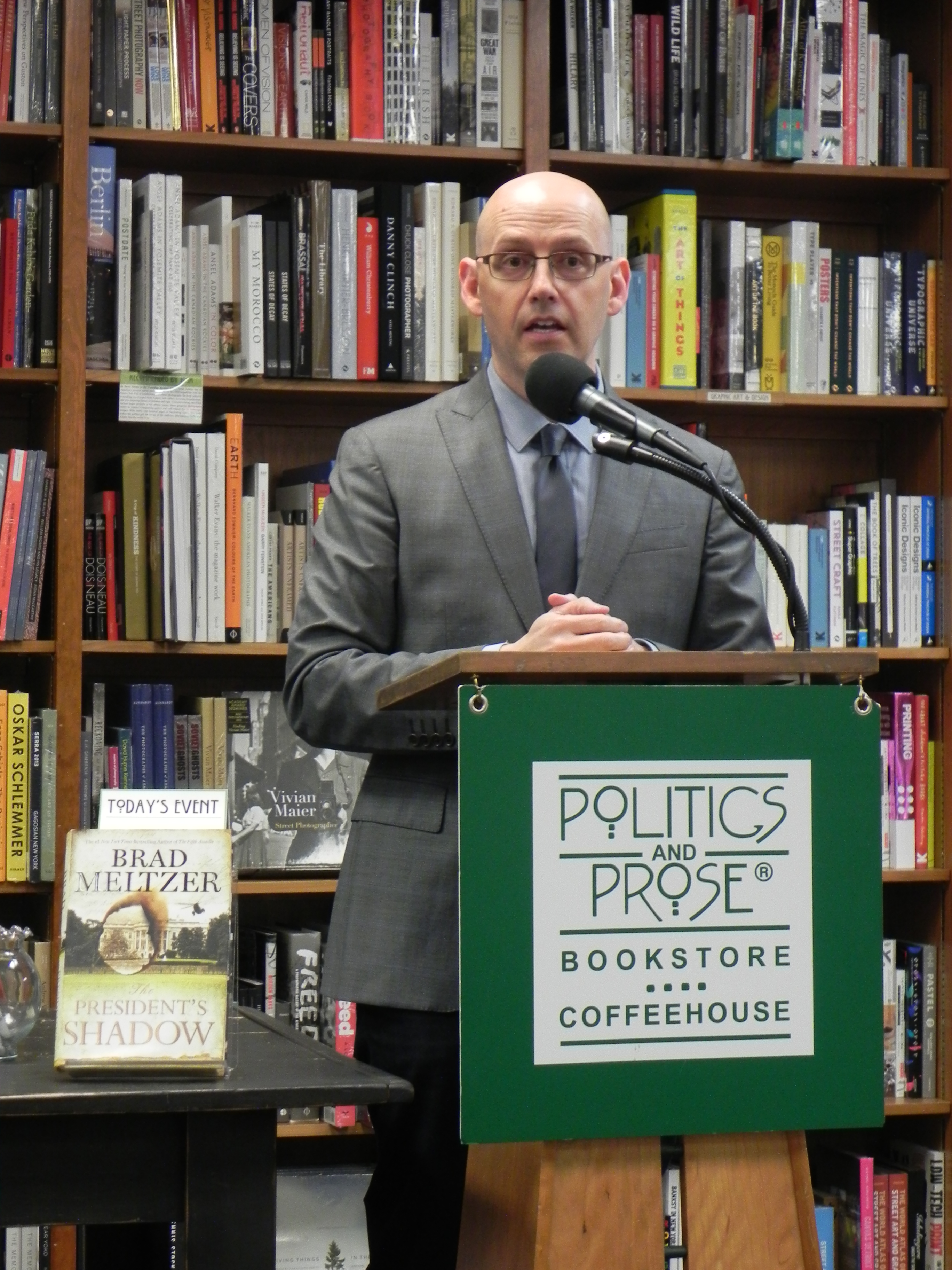In this photograph, a bald man with round glasses is standing behind a brown wooden podium, in what appears to be an indoor bookstore or coffeehouse setting. The podium has a poster attached to it, displaying the text "Politics and Prose, Bookstore Coffeehouse" in green font on a white background. The man is speaking into two microphones attached to the podium and is dressed in a light blue shirt, a gray coat, a gray tie, and black pants. Surrounding him are five shelves filled with books. To his left, there is a table with a book placed on it. The book, titled "President's Shadow" by Brad Meltzer, has a yellowish cover with some imagery that is difficult to discern, possibly depicting a face with buildings in the background. The setting suggests he is addressing an audience about the book.